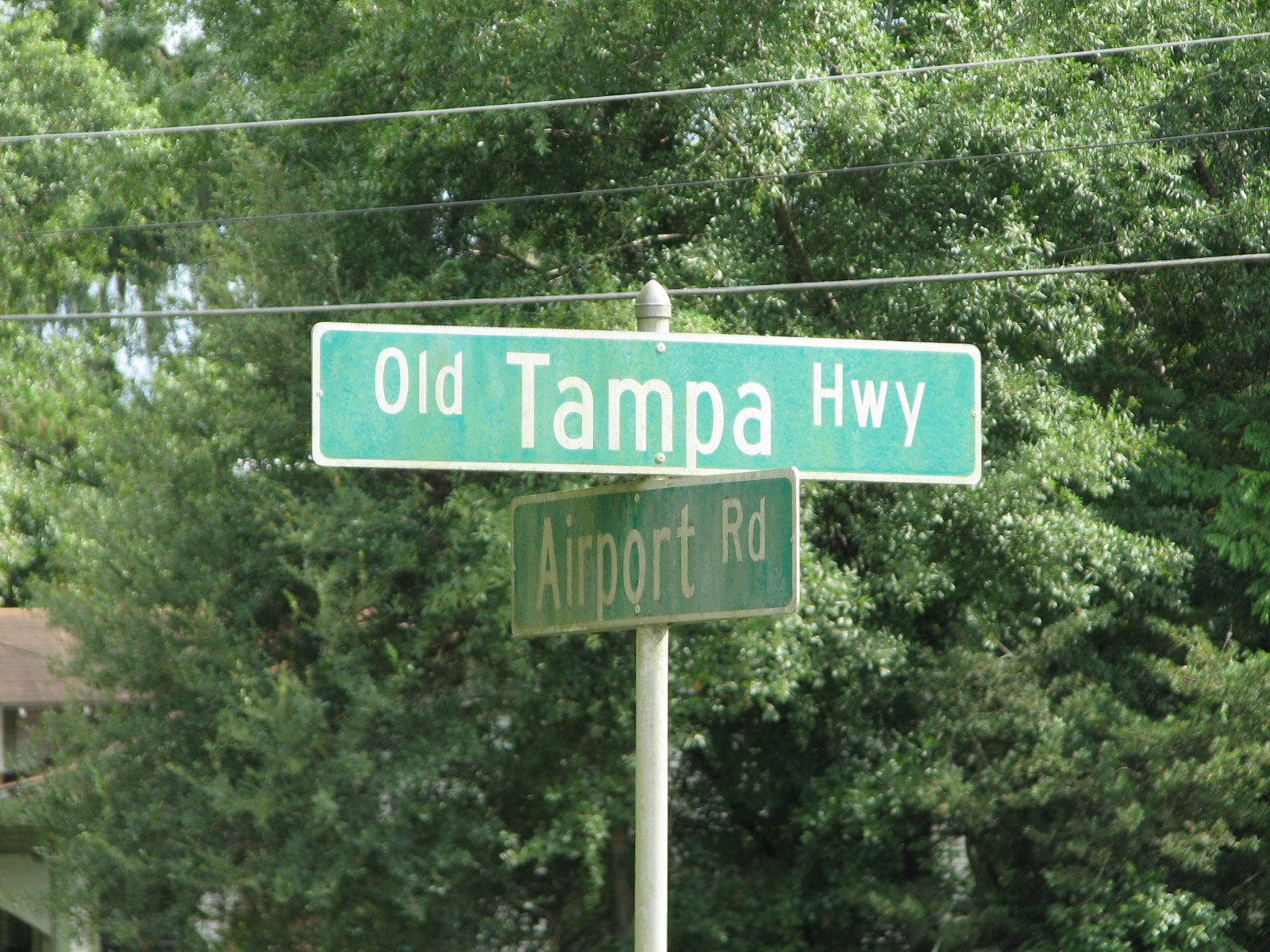This photograph captures a quintessential American streetscape, centered on a prominently featured white signpost that rises from the bottom of the image to about two-thirds of the way up. Mounted on the post are two rectangular, green street signs with white text. The sign facing directly towards the camera reads "Old Tampa Highway" (abbreviated as "Old Tampa HWY" on the sign), while the other sign, positioned perpendicular to the first, reads "Airport Road" (abbreviated as "Airport RD"). Above the signpost, three electrical wires—two thick and one thin—stretch across the image. In the bottom left corner, the brown roof and white wall of a house are partially visible. The backdrop consists of dense, dark green bushy trees, enveloping the scene in foliage. The photograph distinctly emphasizes the intersection marked by these street signs, evocative of American suburban or rural environments.